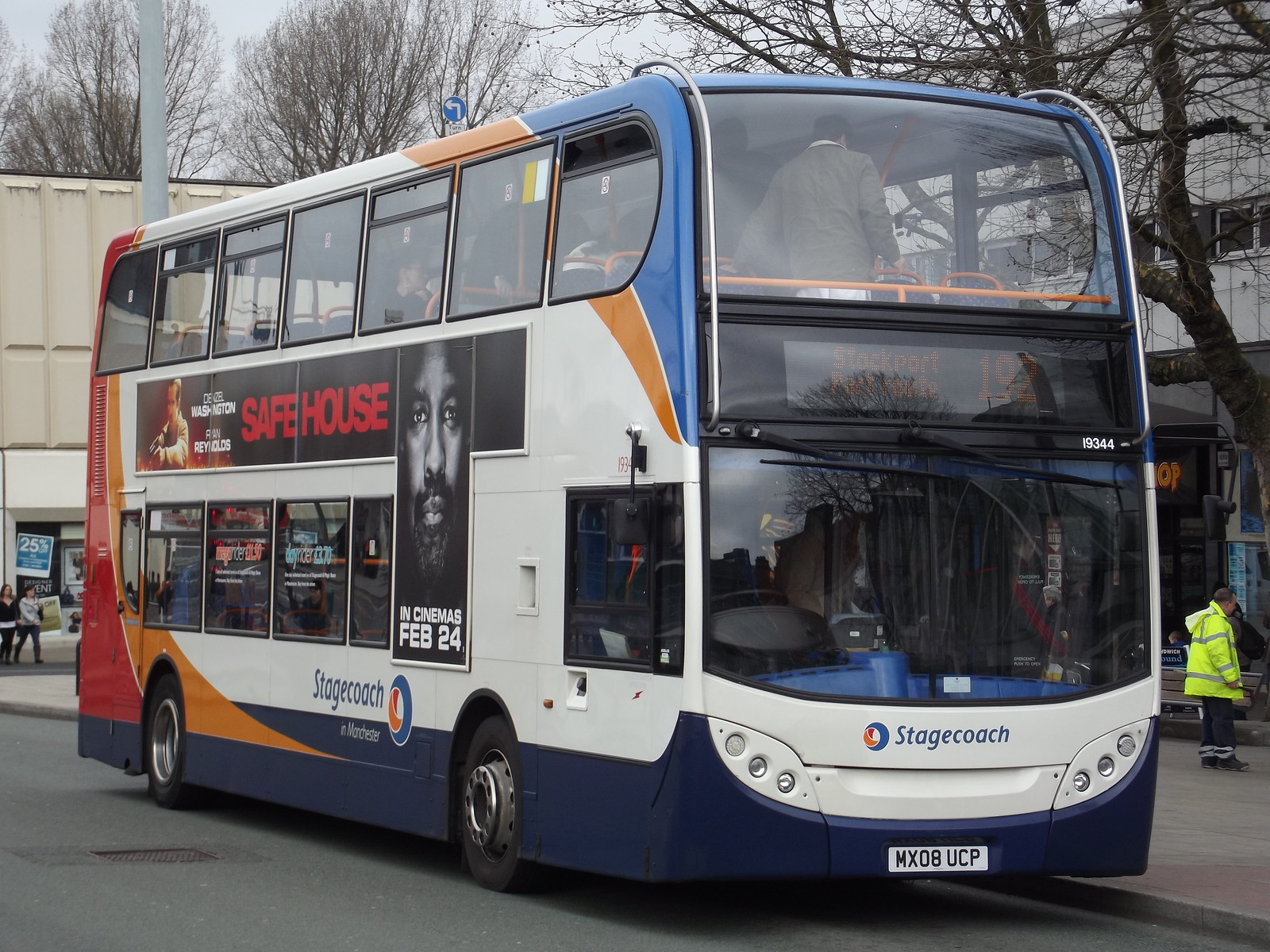This daytime outdoor photograph captures a double-decker bus parked along a city street, with a detailed backdrop of an urban setting featuring a store wall and leafless trees, suggesting fall or winter. The bus, operated by Stagecoach, is predominantly white with distinct blue, orange, and red borders on the front and back. The Stagecoach logo is prominently displayed on both the front and side of the bus. The bus features multiple advertisements; most notably, a large poster for the movie "Safe House" starring Denzel Washington and Ryan Reynolds, set to release in cinemas on February 24th. The vivid movie poster expands along the side of the bus, with Ryan Reynolds' character holding a gun and Denzel Washington’s face prominently displayed in black and white. Other smaller ads are also present but are too distant to decipher. Standing to the right of the bus is a person in a fluorescent green jacket with reflective tape, likely a city worker. Inside the bus, passengers are visible on both levels, adding to the bustling city atmosphere.